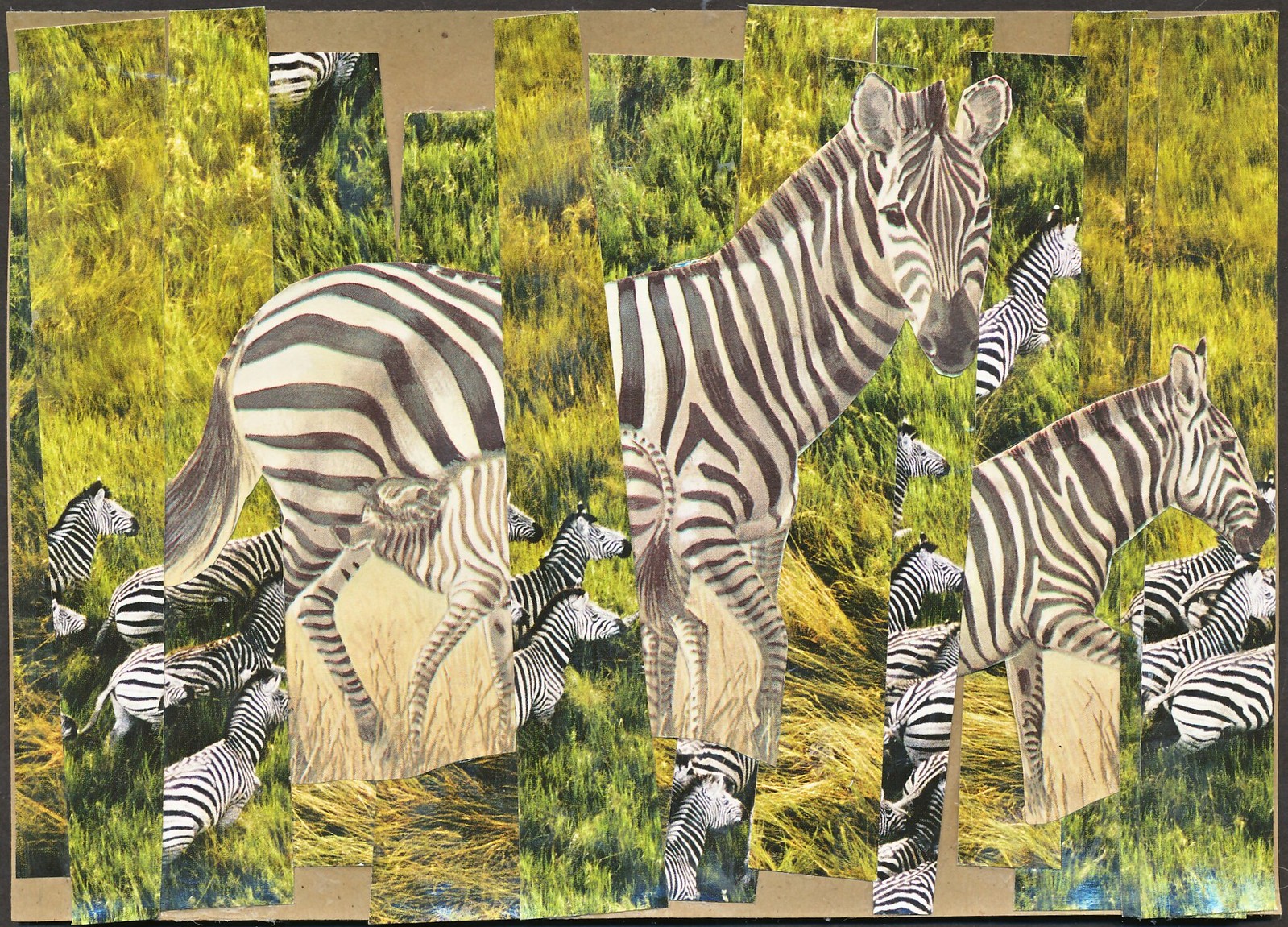The image portrays a meticulously assembled art piece featuring zebras in a grassy plain. This piece is composed of several uneven, thin strips cut from a photograph and pasted onto a brown cardboard background. The strips are misaligned, creating a disjointed, puzzle-like effect. Prominently, there's a large zebra taking up the center of the image, with visible back legs and a missing tail tip. This central zebra, seemingly either photographic or illustrated, draws most attention. In the background, additional zebras, possessing a less distinct black and white coloration, are scattered across the strips, some of which are shorter and further misaligned, resulting in fragmented zebra figures. These zebras appear to be in different positions and orientations, enhancing the collage's dynamic nature. The grass varies in height and color - taller and greener at the bottom and more tan and dry towards the top, contributing to the sense of depth. This artistic representation, set under daylight with visible shadows, gives an impression of both chaos and unity in a sunlit, expansive grassy plain.